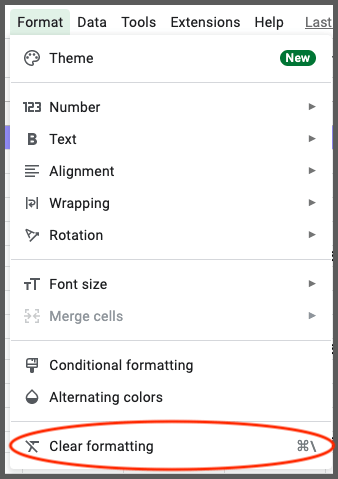The image appears to be a screenshot of a settings menu, potentially within a text document or spreadsheet application. At the top left corner, there is the word "Format" highlighted with a light greenish background within a rectangular box. Horizontal to the right, the menu continues with the words "Data," "Tools," "Extensions," "Help," and "Last." The word "Last" is located at the top right corner and is underlined in a light gray color.

On the far left, at the top, there is a vertical list starting with the word "Theme," which is accompanied by a small pink canvas icon to its left. Below "Theme," the list continues with "Number," followed by the numbers "1, 2, 3" to the left of it. Further, the list includes "Text," "Alignment," "Wrapping," "Rotation," "Font Size," "Merge Cells," "Conditional Formatting," "Alternating Colors," and "Clear Formatting."

To the left of "Text" and proceeding downwards, there are icons such as a bold "B," some lines, and to the right of "Number," "Text," "Alignment," "Wrapping," "Rotation," "Font Size," and "Merge Cells," there are small arrows pointing to the right.